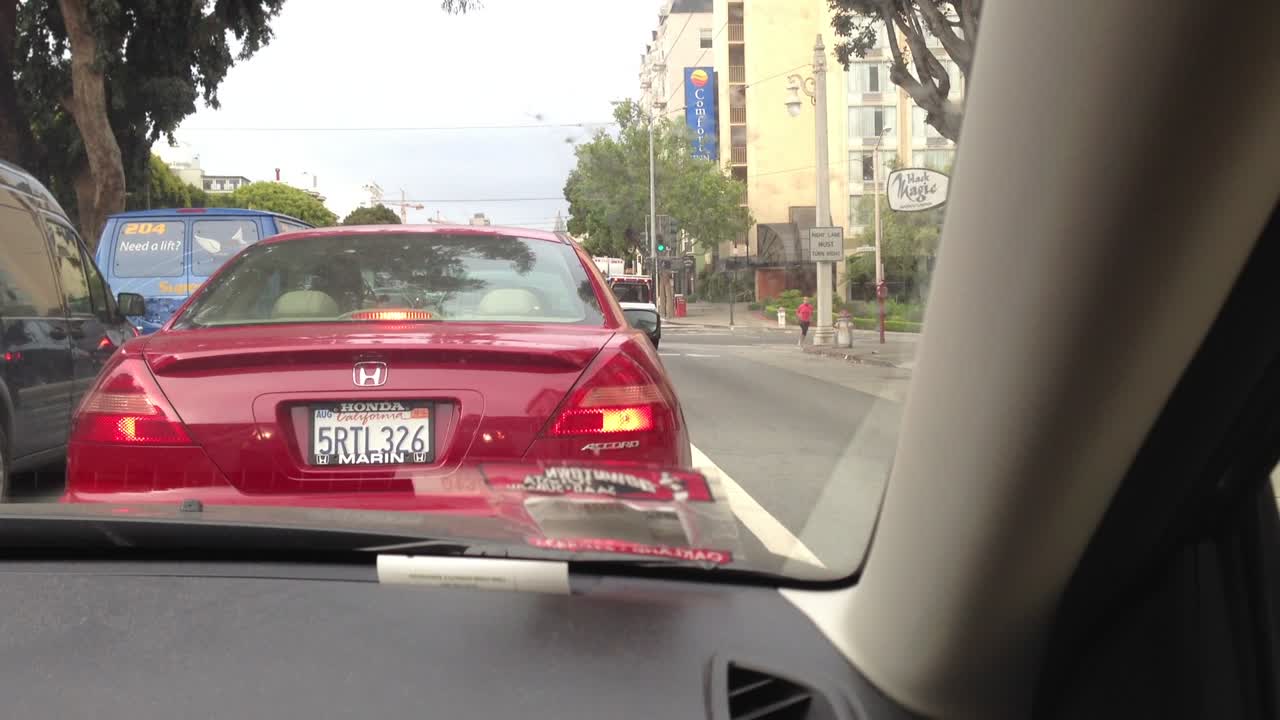This color photograph, taken from the passenger side of a vehicle driving down a busy street, captures a moment in various traffic. Directly ahead is a maroon Honda Accord with the license plate 5RTL326, its brake lights glowing red. In front of the Honda is a black mini pickup, while in the left lane, alongside these vehicles, are a dark blue or black minivan and a blue regular van displaying a yellow "204" and "SIG" in white lettering. The van bears the words "need a lift" in white. To the right, the store "Mask Magic" is visible, marked by its white sign stating "Right Lane Must Turn Right." Nearby is a jogger in a red shirt and black tights, nearing the corner. Further down the block, a Comfort Inn hotel and a green traffic light are discernable. The cityscape features tall buildings with balconies, electric lines crossing the sky, and lush trees lining both sides of the street, including one particularly large tree on the left. On the vehicle's dashboard, a receipt is casually placed, adding a personal touch to the scene.